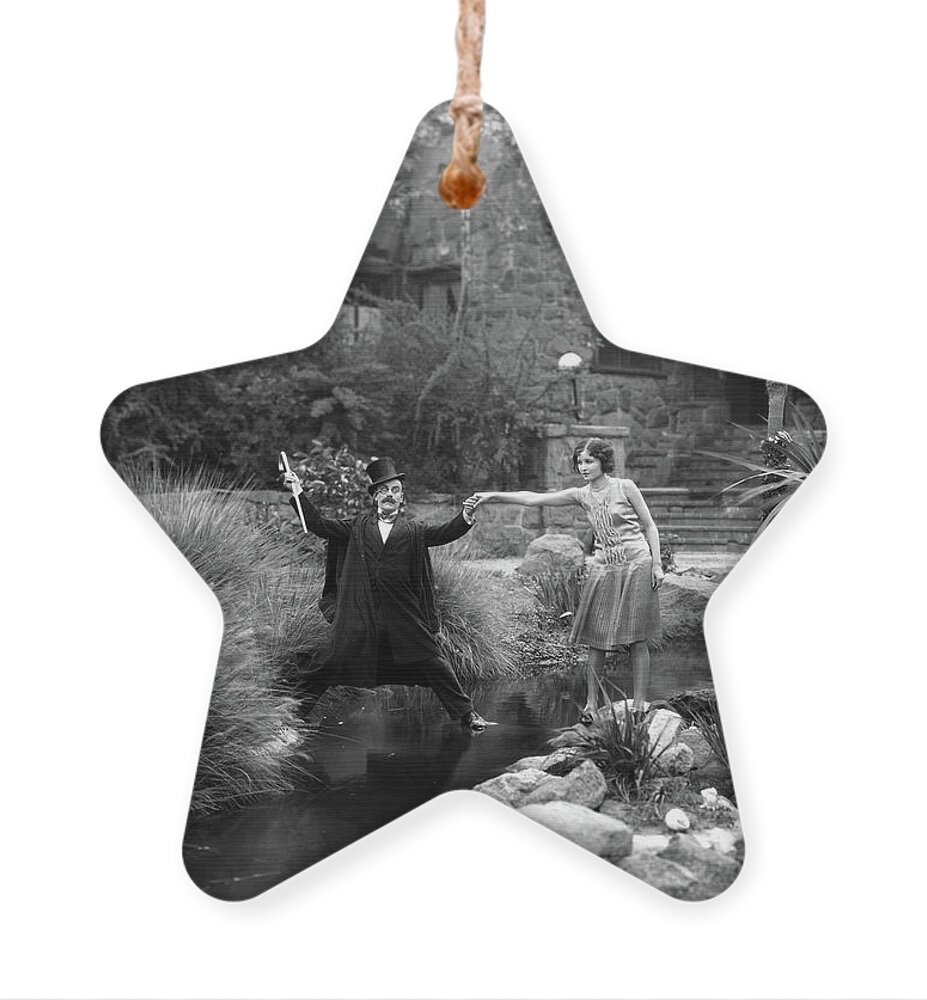This black and white image, likely dating from the 1920s and designed to be a decorative ornament or house decoration, depicts a poignant scene outside a multi-story stone house. The well-dressed man in a top hat and black suit, holding a cane, tentatively balances with one leg hovering over a quaint water feature, as he attempts to cross. Opposite him, a woman, already on the other side, holds his hand to assist him in his crossing, providing a sense of companionship and care. Her posture suggests determination as she helps prevent him from stumbling. In the background, the stone facade of the house and a set of stairs leading up to it add to the charming, historical appeal of the photograph. The image resonates with an old-world charm, capturing a moment of tender human interaction against a backdrop that suggests an era where such scenes were commonplace.